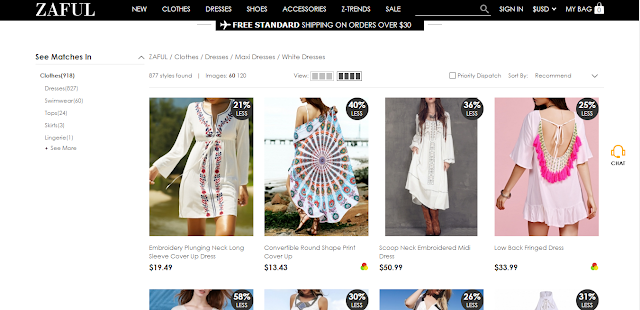This horizontally-oriented image appears to be a screenshot from a women's clothing website, specifically showcasing the Zaful online store. The background is predominantly white, offering a clean and minimalist look typical of many e-commerce sites.

At the very top of the image, there is a bold black bar. In the upper left-hand corner, the site name "ZAFUL" is prominently displayed in uppercase white letters. The navigation menu follows, also in white text, with options arranged from left to right: New Clothes, Dresses, Shoes, Accessories, Z-Trends, Sale. Further to the right, there is a magnifying glass icon for the search bar, a currency selection labeled "USD," and an icon resembling a shopping bag currently showing zero items inside.

Beneath this navigation bar, a banner promotes free shipping on orders over $30. The banner text invites you to explore various categories, such as Clothes, Dresses, Swimwear, Tops, Skirts, and Lingerie, with a "See More" option available.

Further down, the image highlights a breadcrumb navigation trail, which reads: Zaful / Clothes / Dresses / Maxi Dresses / White Designs. Alongside, it displays the number of items found, the view mode, dispatch details, and sorting options like "Sort by Recommend." Following this, the image transitions into showcasing photographs of a woman modeling various dresses that meet the search criteria, each elegantly styled to entice shoppers.

The structured layout and comprehensive features aim to provide an intuitive and user-friendly shopping experience.